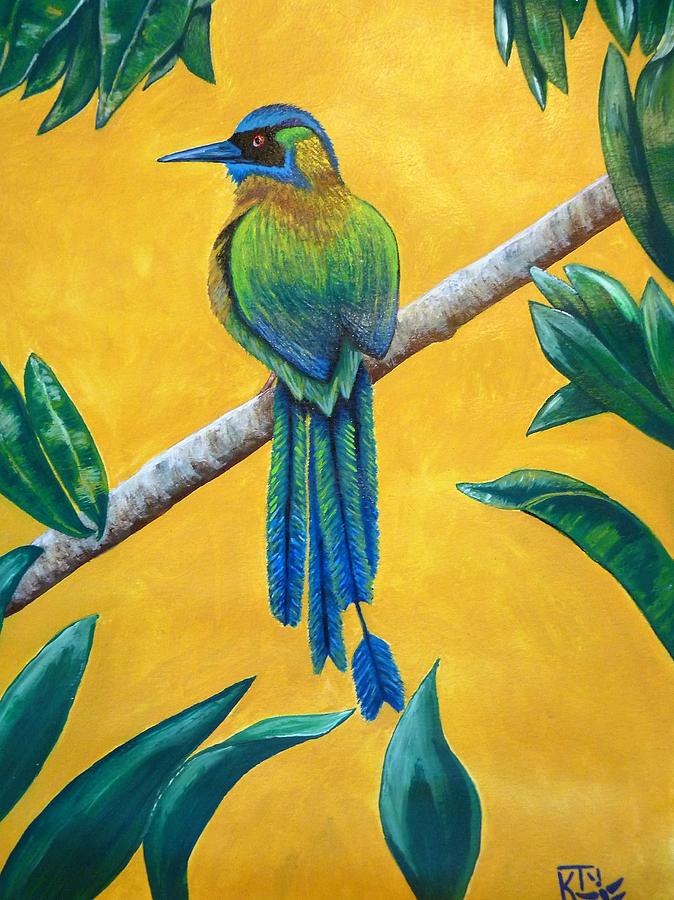The image showcases a beautiful drawing signed with what appears to be either the initials "K and Y" or a "K" accompanied by an insect illustration, though the exact signature remains ambiguous. The background of the artwork is a rich, dark gold, creating a striking contrast with the foreground elements. A light brown branch spans diagonally from the lower left to the upper right of the composition, providing a perch for a stunning medium bright blue bird. 

This bird has a vibrant bright blue beak, head, tail feathers, and wing tips. Its eyes are surrounded by a ring of black, blending into its amber irises, which in turn encircle the black pupils. The area around the eyes also features soft touches of lighter green and gold. The bird's wings are accented with lighter green, adding depth and variety to its plumage. The drawing includes large green leaves, some of which transition to a blue hue, particularly at the bottom, possibly due to lighting effects or artistic interpretation. The leaves at the top retain their green coloration, subtly tinged with blue, harmonizing with the overall color scheme of the artwork.